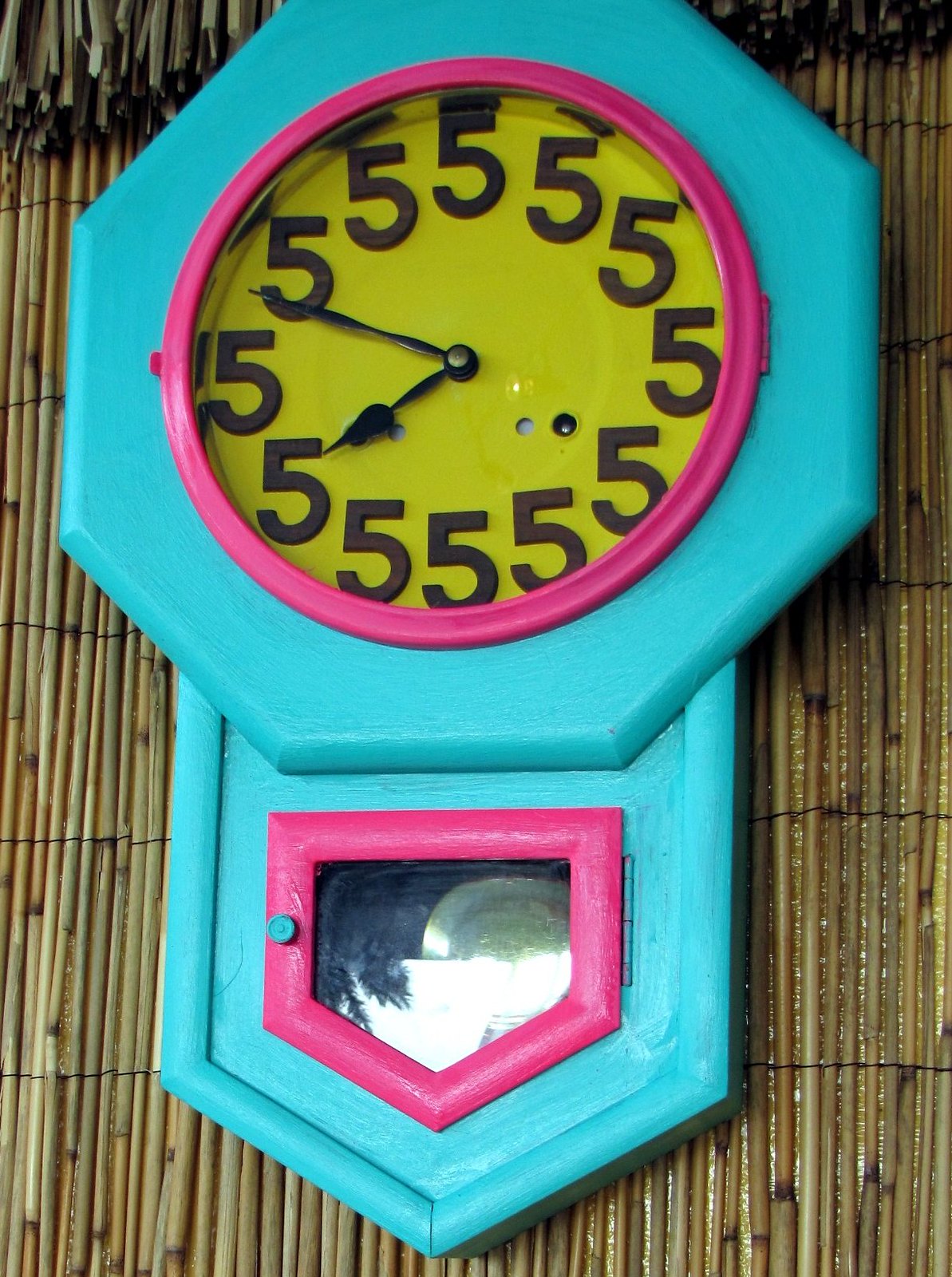This vibrant and whimsical wall clock, crafted from wood, boasts a playful design with its octagonal shape. Painted in a bright turquoise, it features trim pieces in a neon-like dark pink, adding a striking contrast. The clock face, uniquely painted in yellow, breaks tradition by displaying the number five in place of all other numerals, encircling its entirety. The hour and minute hands stand out in bold black, providing clear visibility. Below the clock face, a small trap door reveals a hint of a pendulum, further enhancing its eccentric charm.